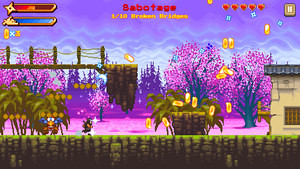The image appears to be a detailed scene from an older, pixelated video game, likely from the eighties or early nineties, with unsophisticated graphics. The landscape-oriented scene features several notable elements: across the bottom is a dark stone wall, with green bushes growing behind it and bright pink, fuchsia-colored ground. Purple trees with blue limbs and bright pink leaves adorn the background, creating a colorful, whimsical environment. 

A character, possibly a man, is depicted sprinting with sparkles around his head, accompanied by a small, colorful blue bird with a yellow beak. There is a half-completed log bridge extending from the left side of the image, which ends abruptly, creating a potential cliff.

To the right of the scene is a house with white walls, a blue roof, and windows, surrounded by purple trees and flowers. Scattered gold coins suggest an interactive or collectible element in the game. Several interface elements enhance the game's visual context: hearts in the right-hand corner indicating life or love for the game, and a red bar with a ninja shuriken at the top left, next to a sliding symbol. 

The sky above is a textured blue, featuring a playful tone reminiscent of early video game aesthetics. At the top of the screen, red text reads "Sabotage" with a subtitle in yellow stating "1/10 Broken Bridges," suggesting a level or mission objective. Overall, the scene captures the essence of nostalgic digital adventures with a vibrant and engaging environment.